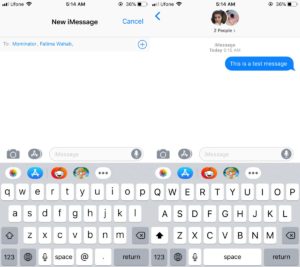This image is a blurred and small screenshot displaying a text messaging interface. The top section indicates it is a new iMessage conversation involving three participants. A blue dialogue bubble conveys the message, "This is a test message." Positioned at the bottom, the keyboard is visible, displaying lowercase letters in the traditional QWERTY layout on the left, and on the right, a similar keyboard layout but featuring all capital letters. Above the keyboard, several icons are discernible though details are unclear due to the image quality. The dimensions of the image appear nearly equal both horizontally and vertically. Notably, the image lacks any visual presence of people, animals, plants, or objects such as motorcycles or bicycles.